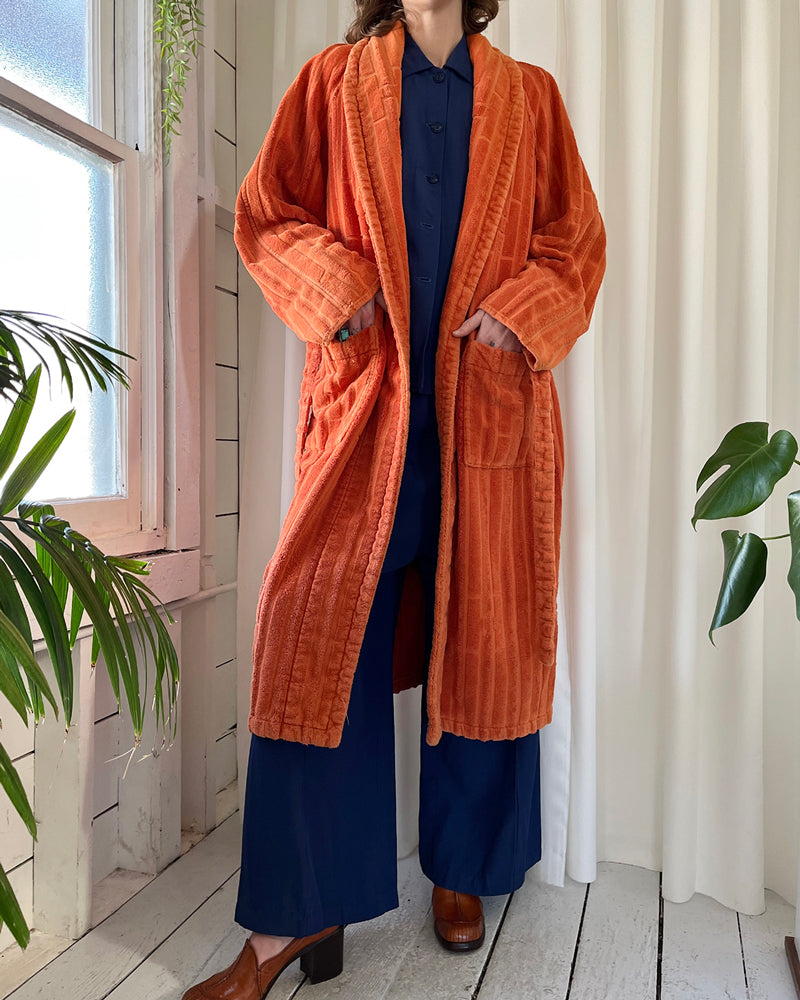The photograph portrays a woman standing in the center of what appears to be a bathroom with a rustic aesthetic. The floor and walls are constructed from wooden planks, painted a white or grayish-white that leaves the natural texture visible. There are visible gaps between some planks, enhancing the rustic, almost cabin-like feel. She stands amidst this setting, framed by flowing white curtains and surrounded by green houseplants positioned to her sides and slightly behind her. A window with a white-painted frame is discernible on the left side of the image.

The woman is dressed in a striking combination of a formal and casual outfit. She wears a blue button-up jumpsuit or pantsuit paired with a cozy, fuzzy orange robe draped over it. Her footwear consists of chunky, wooden-colored leather high heels. She strikes a model-like pose, exuding an air of calm sophistication. Her hands are casually tucked into the pockets of her robe, with a hint of a ring visible on her right hand. The overall composition conveys a blend of comfort and elegance, set against the backdrop of a tastefully decorated rustic room.